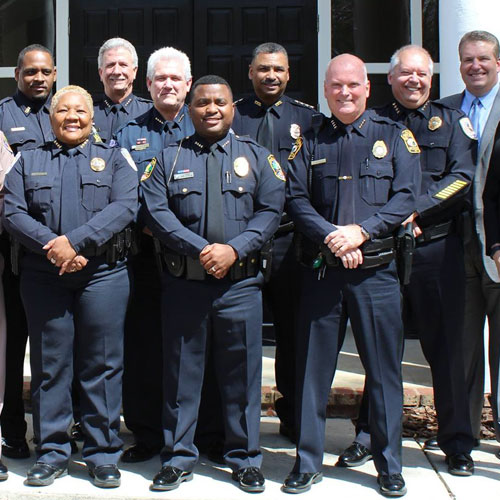In this outdoor photograph, a group of nine police officers, comprising multi-racial members including Caucasian and Black men, and one Black woman, are posing in front of a building with visible black doors. Eight of them are dressed in deep navy blue uniforms complete with matching navy blue ties, shiny black boots, and black belts equipped with various accessories and firearm holders. They display their golden police badges prominently on their right chest and sleeves. The officers stand with their feet slightly apart and their hands clasped in front of them, looking directly at the camera with pleasant smiles, indicative of their camaraderie and pride. Interestingly, there is one Caucasian man on the far right who stands out in a gray suit coat, adding a unique element to the otherwise uniformed group.